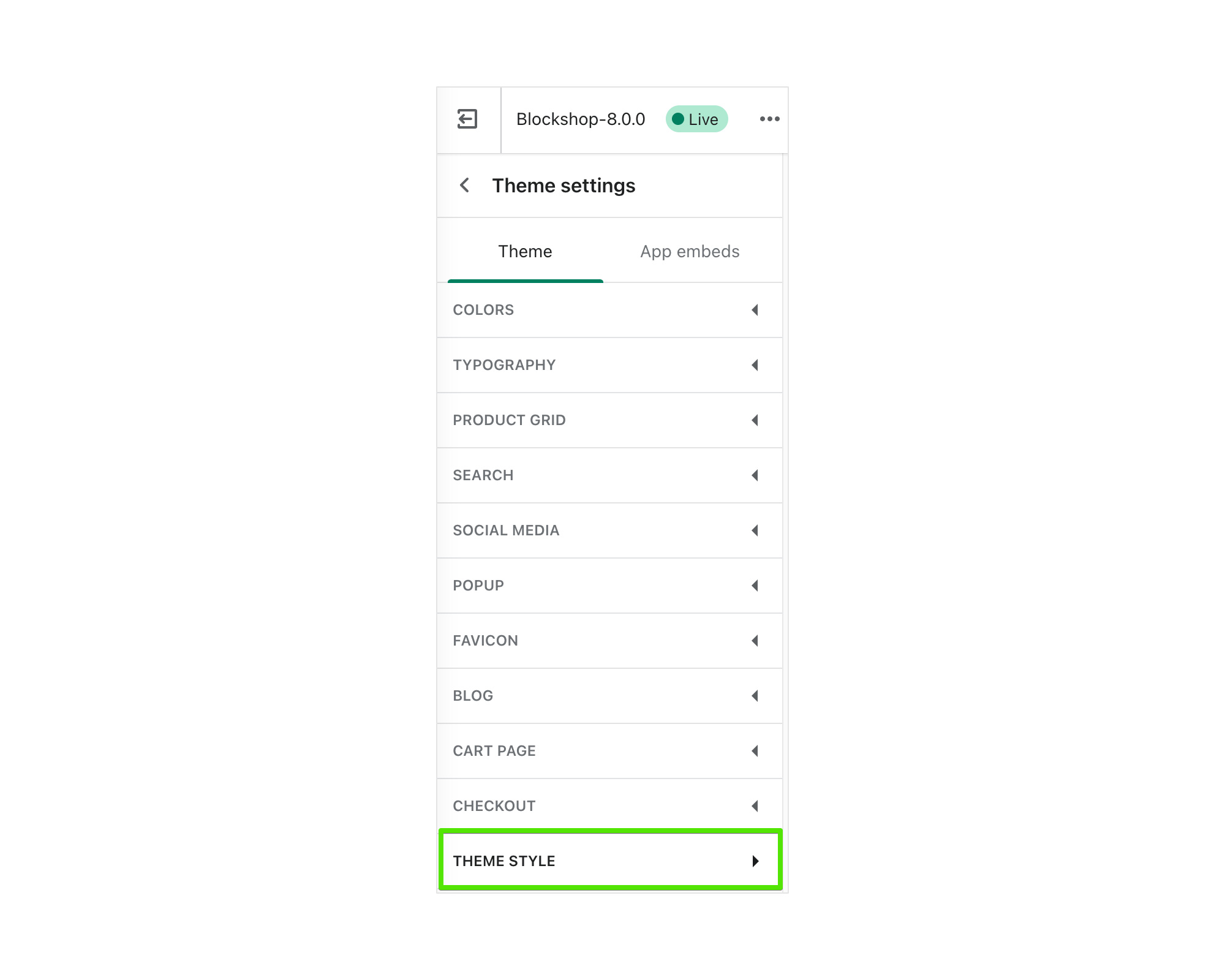The image showcases a settings menu interface on a digital platform, titled "Blockshop - 8.0.0 live." The menu is displayed within a white box that does not occupy the full screen but a portion of the background space. At the top, there is a left-pointing arrow, followed by the title "Blockshop - 8.0.0 live," and a hamburger menu icon.

Below this header, the interface is divided into distinct sections. The first section is labeled "Theme Settings," accompanied by a left-pointing arrow. Under this, two subheadings read "Theme" and "App Embeds."

Following these subheadings is a vertical list of settings options, each with a left-pointing arrow aligned to the right. The options are:

1. Colors
2. Typography
3. Product Grid
4. Search
5. Social Media
6. Pop-up
7. Favicon
8. Block
9. Cart Page
10. Checkout
11. Theme Style

The "Theme Style" option stands out as it is not only written in uppercase like the others but is also bold and highlighted with a lime green bar. Additionally, the arrow next to "Theme Style" points to the right, differentiating it from the left-pointing arrows used for the other options.